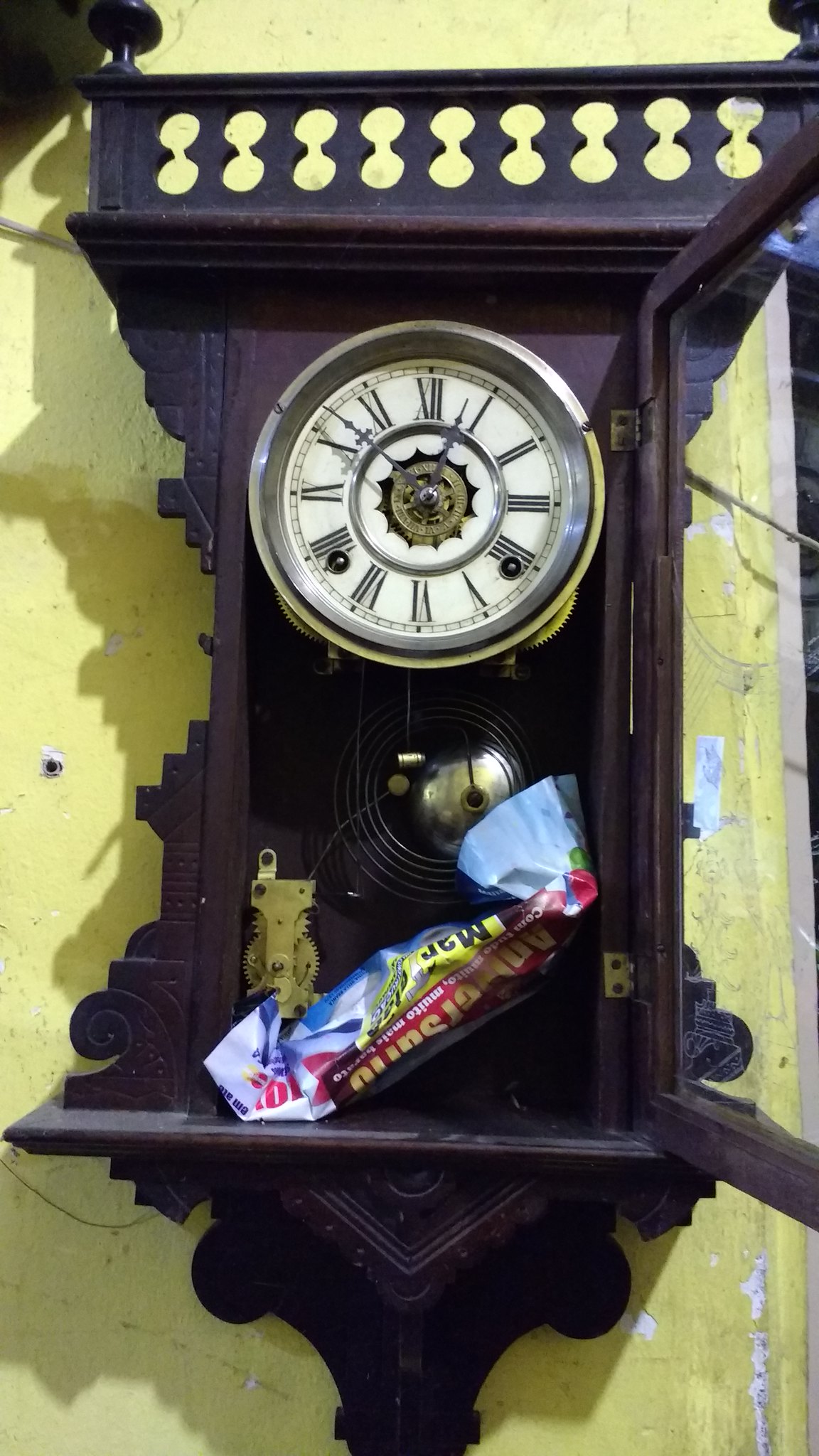The image showcases an antique pendulum-style wall clock mounted on a weathered yellow wall with peeling paint and random dirty tape marks. The clock features an ornate wooden case in a dark finish, adorned with intricate jigsaw-style woodwork and curly Q's. Its design includes a brown latticework panel at the top and a fleur-de-lis-like pattern at the base. The clock has a white face with Roman numerals I through XII, and black ornate hour and minute hands. There are two winding holes and a brass ring at the center. The clock's glass door is ajar, revealing visible internal gears and mechanisms typically hidden. Inside, a rolled-up piece of paper or possibly a candy bar wrapper in blue, white, yellow, and red is wedged, suggesting the clock might be under repair. The unusual state of the clock coupled with its broken, aged surroundings gives the entire scene a sense of dilapidated charm and history.